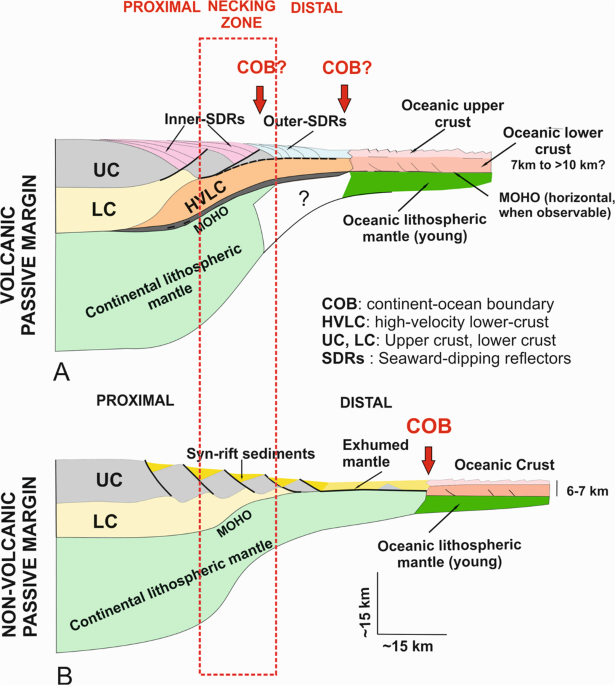The image is a detailed geological diagram featuring a cross-section of volcanic and non-volcanic passive margins. At the top, prominent red text labels the "Proximal Necking Zone" and "Interstitial Zone," with a red-dotted rectangle outlining the necking zone across both diagrams. To the left, black text identifies "Volcanic Passive Margin" and "Non-Volcanic Passive Margin" corresponding to diagrams A and B, respectively. The intricate cross-sections, resembling the shape of Idaho on its side, depict multiple earth layers labeled with abbreviations. A legend in the center explains these: UC (Upper Crust), LC (Lower Crust), HVLC (High-Velocity Lower Crust), SDR (Seaward Dipping Reflectors), and COB (Continent Ocean Boundary). The continental lithospheric mantle is noted across the bottom, providing a comprehensive technical illustration of these geological features.